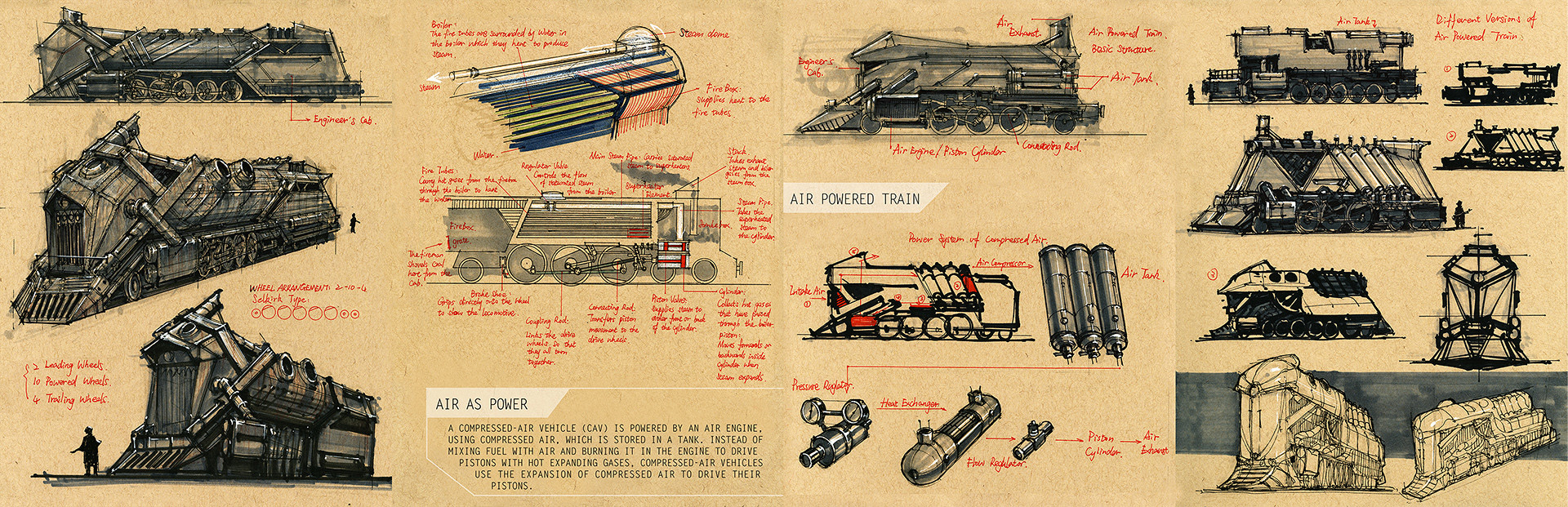The image is a detailed, informative illustration primarily focused on air-powered trains. The rectangular plaque, about six inches wide and one and a half inches tall, is sectioned into four columns. The background is a light brown, almost tan, color. 

In the first column on the far left, there are three vertically aligned drawings of locomotives, each with red print underneath pointing to various parts of the trains. 

The second column features a side view of a train with numerous red lines and annotations indicating different components of the locomotive. This section is rich in text, including a paragraph explaining how a compressed air vehicle (CAV) operates. It elaborates that a CAV uses compressed air stored in a tank to power an engine, driving pistons through the expansion of this air rather than combustion.

The third column includes another side view of the train with additional detailed annotations. It prominently displays the text "air-powered train" on a white background with black lettering.

In the fourth and final column, there are more schematic drawings of the trains from various angles, with red text pointing out specific parts. This section provides a comprehensive visual summary of the locomotive designs for compressed air vehicles, emphasizing the mechanics and structure of air-powered trains.